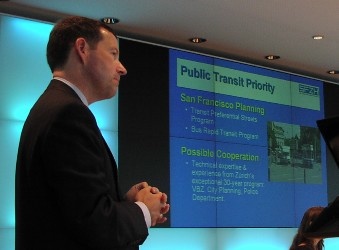The image depicts a man, likely a speaker or lecturer, standing with his hands folded in front of him. He is dressed in a dark suit with a white shirt, and has short brown hair and fair skin. The man is situated to the left side of the image, appearing to listen attentively, possibly to someone else who is speaking. Behind him, a blue wall is illuminated, featuring a recessed black screen that displays a presentation slide. The slide has a blue background with yellow and white text, reading "Public Transit Priority" at the top, and further detailing aspects of "San Francisco Planning" related to bus rapid transit and possible cooperation. The text includes phrases such as "Technical Expertise," "VBZ City Planning Department," and references to cooperation and an exceptional 30-year program. The slide also includes a small image of two vehicles, likely buses, on a city street. The room's ceiling is white with some recessed lights, many of which are turned off. In the bottom right corner of the image, partially obscured by a black object, the head of a woman with long brown hair is visible, suggesting the speaker is addressing an audience.